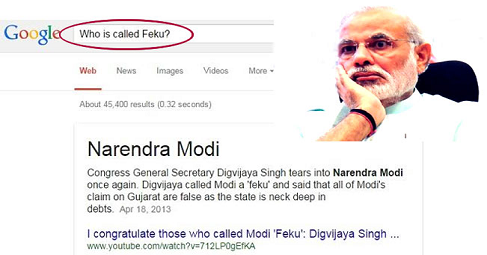Here is the revised and detailed caption for the described image:

---

The image is a small screenshot captured in landscape orientation, seemingly from a Google search results page. In the upper left-hand corner, the familiar Google logo is displayed alongside the search query: "Who is Feku?" The term "Feku," spelled F-E-K-U and followed by a question mark, is circled in red, drawing attention to the search query. 

Below this, the interface displays five navigational tabs, including "Web," "News," "Images," "Videos," and "More," with the "Web" tab being highlighted in red and underlined, indicating the active search filter. The search results reveal approximately 45,400 results, retrieved in 0.32 seconds.

Positioned in the upper right section of the screenshot is an image of Narendra Modi, the Prime Minister of India. He is an Indian male characterized by a white mustache and beard, balding head, and wire-rimmed glasses. Modi appears contemplative, with his right hand resting against his chin, and he is wearing a black bracelet on his right wrist.

The main content of the screenshot is a news snippet referencing Narendra Modi. It includes a statement from Congress General Secretary Digvijaya Singh, criticizing Modi. The text reads: "Narendra Modi, Congress General Secretary Digvijaya Singh tears into Narendra Modi once again. Digvijaya calls Modi a Feku and said that all of Modi's claims on Gujarat are false as the state is neck-deep in debts." A quoted link appears at the end, saying: "I congratulate those who called Modi Feku," attributed to Digvijaya Singh.

---